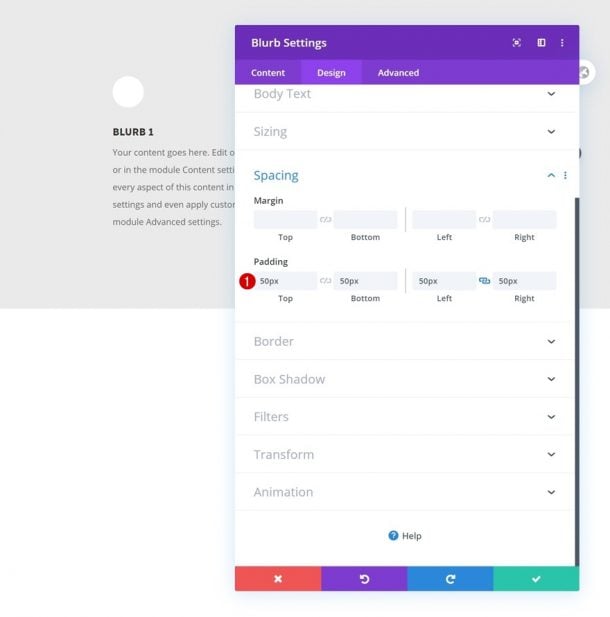The image depicts a user interface featuring a grey background with a title text, "Blurb One," situated beside a white circle. At the top of the screen, there's a prominent purple banner labeled "Blurb Settings," beneath which are three headers: "Content," "Design," and "Advanced." The "Design" tab is highlighted in a slightly lighter shade of purple, indicating it is currently active.

Under the highlighted "Design" tab, the white section of the screen displays various configurable fields and attributes. The "Body Text" section allows adjustment of sizing and spacing, highlighted in blue. Following this, there is an area to modify "Margin," with input fields for top, bottom, left, and right margins. Next, there is a "Padding" section, where the default values are set to 50 pixels for top, bottom, left, and right margins. A red circle with the number "1" emphasizes the top padding input field.

Further attributes listed are "Border," "Box Shadow," "Filters," "Transform," and "Animation." At the bottom of the screen, there are four colored rectangles: orange, purple, blue, and green, adding a touch of visual organization to the interface.